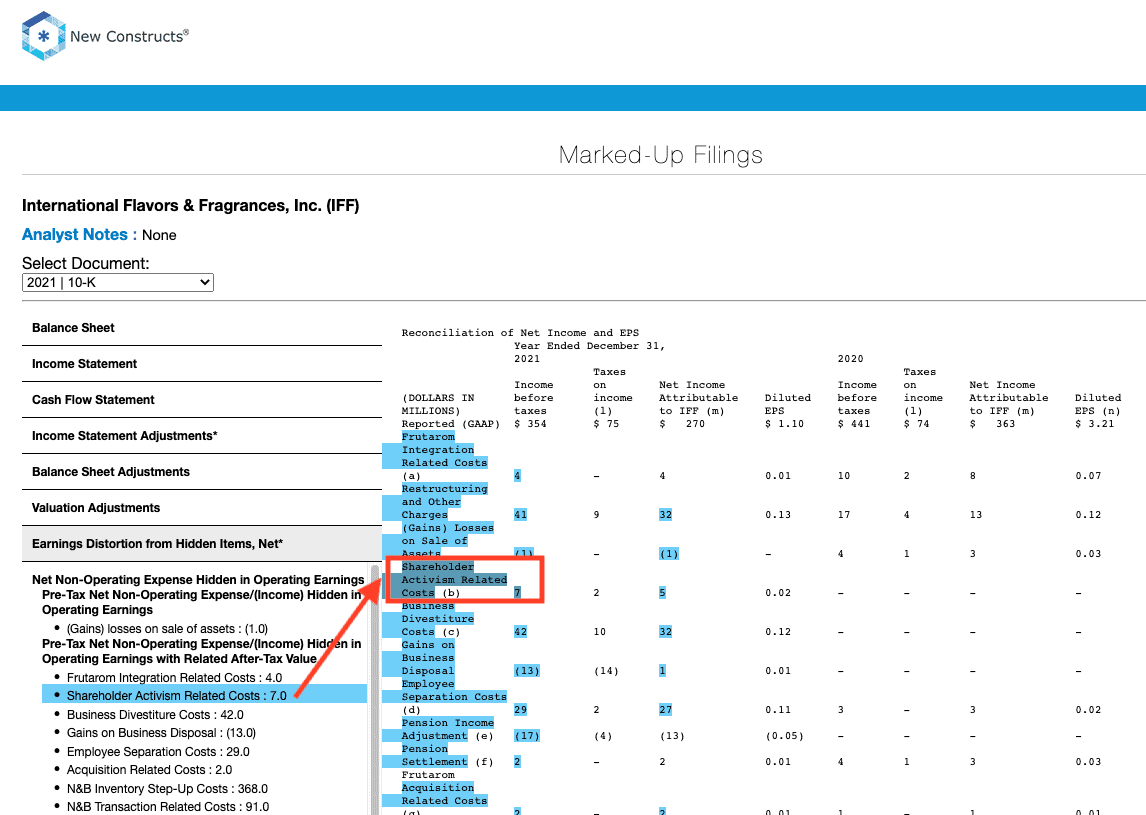The image features a detailed financial document with various annotations and highlights. 

At the top left corner, there is a blue and dark blue octagon with the text "New Constructs." Below this logo, there is a poster followed by a thin blue line. The main content of the image is a report titled "Marked Up Findings," centered at the top in black text. 

On the left side of the report, under the header "International Flavors and Fragrances Inc (IFF)," there is blue text labeled "Analyst Note: None." Further below, black text reads "Select Document: 2021 10-K." The title under this section is "Balance Sheet Reconciliation of Net Income & EPS," which is followed by a detailed table.

The left side menu lists various sections, including:
- Balance Sheet
- Income Statement
- Cash Flow Statement
- Constant Adjustment
- Balance Sheets Adjustment
- Valuation Adjustment

Below these, there's a section titled "Ending Distortion from Hidden Items." This section includes detailed line items with various financial metrics, such as:
- Net non-operating expenses hidden in operating earnings (pre-tax and after-tax values)
- Gains and losses on the sale of assets 
- Integration-related costs: $4.0 million
- Shareholder activism related costs: $7 million
- Business divestiture costs: $42 million
- Employee separation costs: $29 million
- Acquisition-related costs: $2 million
- Inventory step-up costs: $368 million
- Transactional-related costs

"COST: $7 million" is highlighted in blue and pointed out with a red arrow and red outline on the right side of the balance sheet. 

The balance sheet table includes headers such as:
- Millions of Dollars
- GAAP Reported Income Before Taxes
- Taxes on Income
- Net Income Attribute
- Diluted EPS
- Income Before Taxes
- Taxes on Income

The image is a comprehensive, marked-up financial document with clear sections, highlighting hidden costs, and shareholder-related expenses.